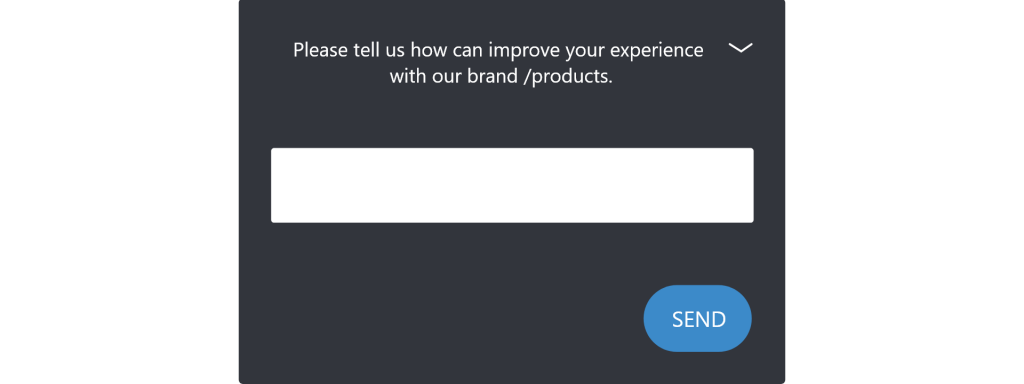The image depicts a rectangular black dialog box that is horizontally oriented. At the center of this black background, the text is center-justified and reads: "Please tell us how we can improve your experience with our brand/products." Immediately next to this text, there's a drop-down menu displayed in white.

Below this prompt, there is a large, bold white data input field. The field appears to be single-line, indicating that users must write their feedback in a continuous line, with no ability to view previously typed text once it exceeds the input field's width.

In the lower right corner of the dialog box, there's a blue button with the word "Send" written in white.

The black dialog box seems to be seamlessly merged with a broader white background, making it appear as a floating element on the predominantly white page. The color scheme is limited to black, white, and blue, with no other colors or elements present in the image.